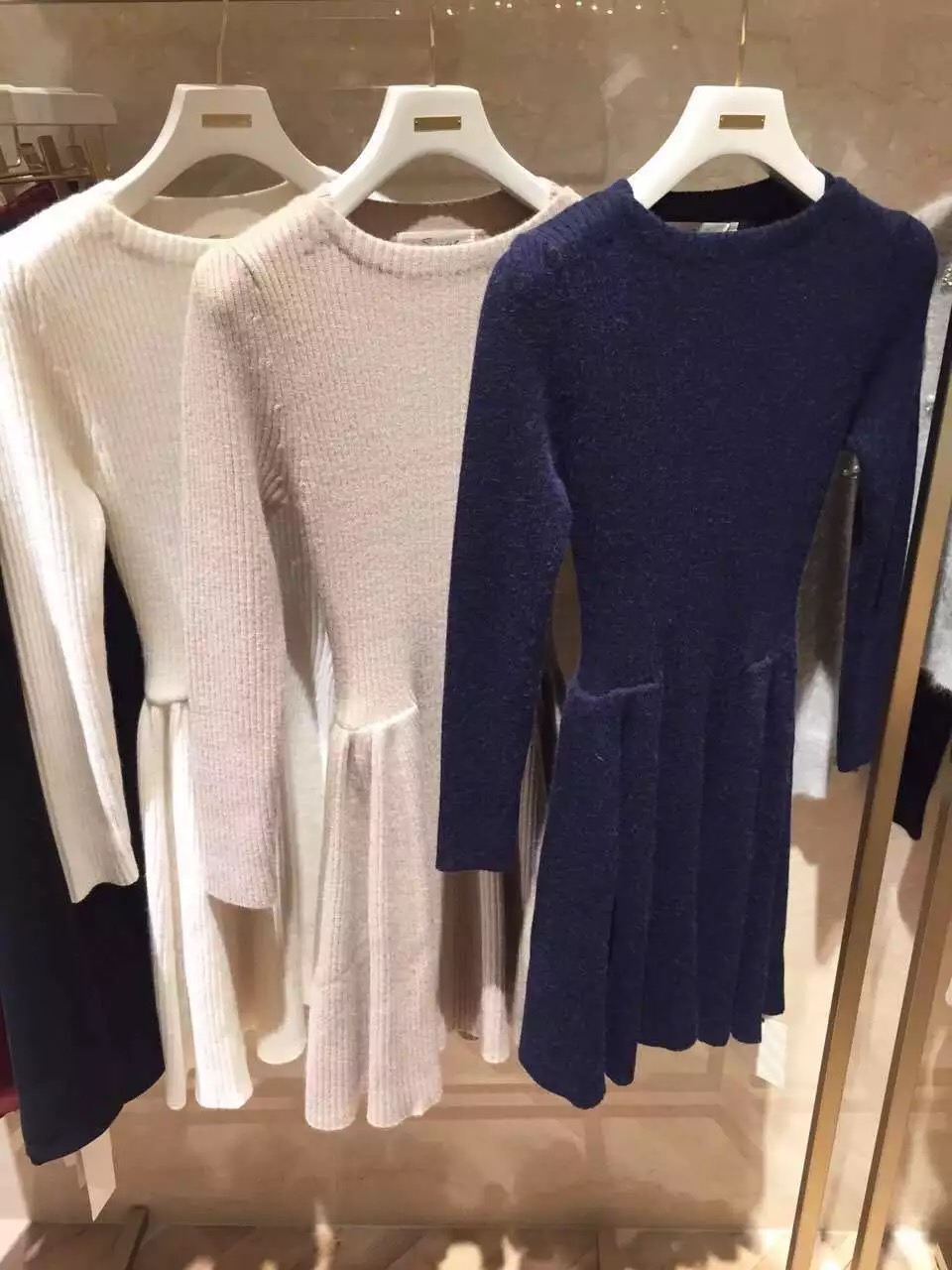In this image, we see three long-sleeved, ribbed sweater dresses hanging from a sleek, gold-colored clothing rack, likely situated in a store due to the glossy, reflective floor. These dresses, made from thick material which could be wool or cashmere, are each suspended on white hangers that feature a distinctive gold strip. The dresses are consistently styled but vary in color: from left to right, they are cream, blush pink, and navy blue. Surrounding the dresses, additional clothing items are partially visible, but remain indistinct in the background. Shadows of the sweater dresses and parts of the clothing rack are noticeable at the bottom of the image, adding depth to the scene.